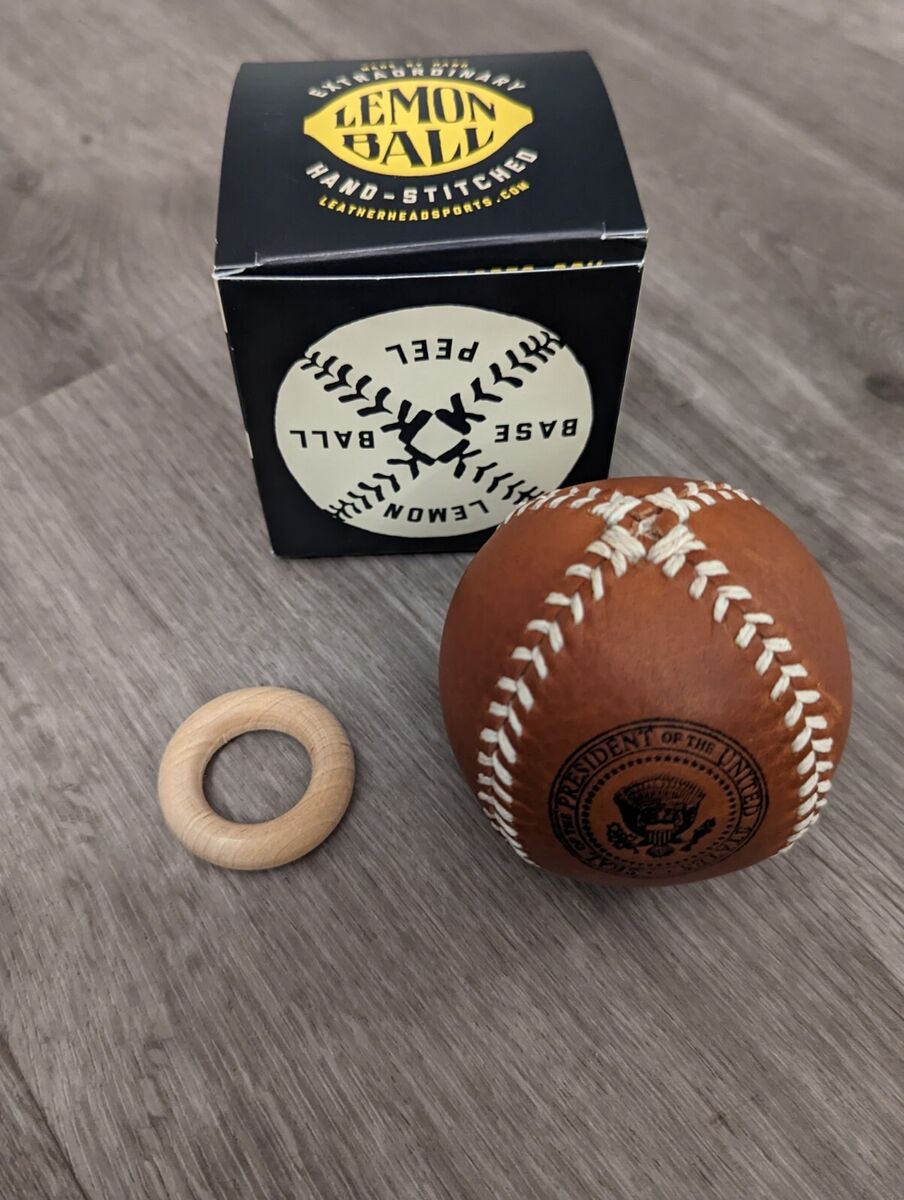The image captures a vintage-esque, dark brown leather ball adorned with white stitching that prominently features the words "President of the United States" and an embossed eagle emblem. Behind the ball is a black box, slightly larger than the ball itself, labeled "Lemon Ball" in white letters and featuring a yellow lemon graphic. This box is inscribed with "hand-stitched" and "leatherheadsports.com" and displays a picture of a white baseball with black stitching labeled "Lemon Peel Baseball" in an X pattern. Additionally, a small wooden ring, possibly included for scale, lies beside the ball. All these items are set against a grayish laminate floor with white stripes, contributing to the overall vintage aesthetic of the scene.